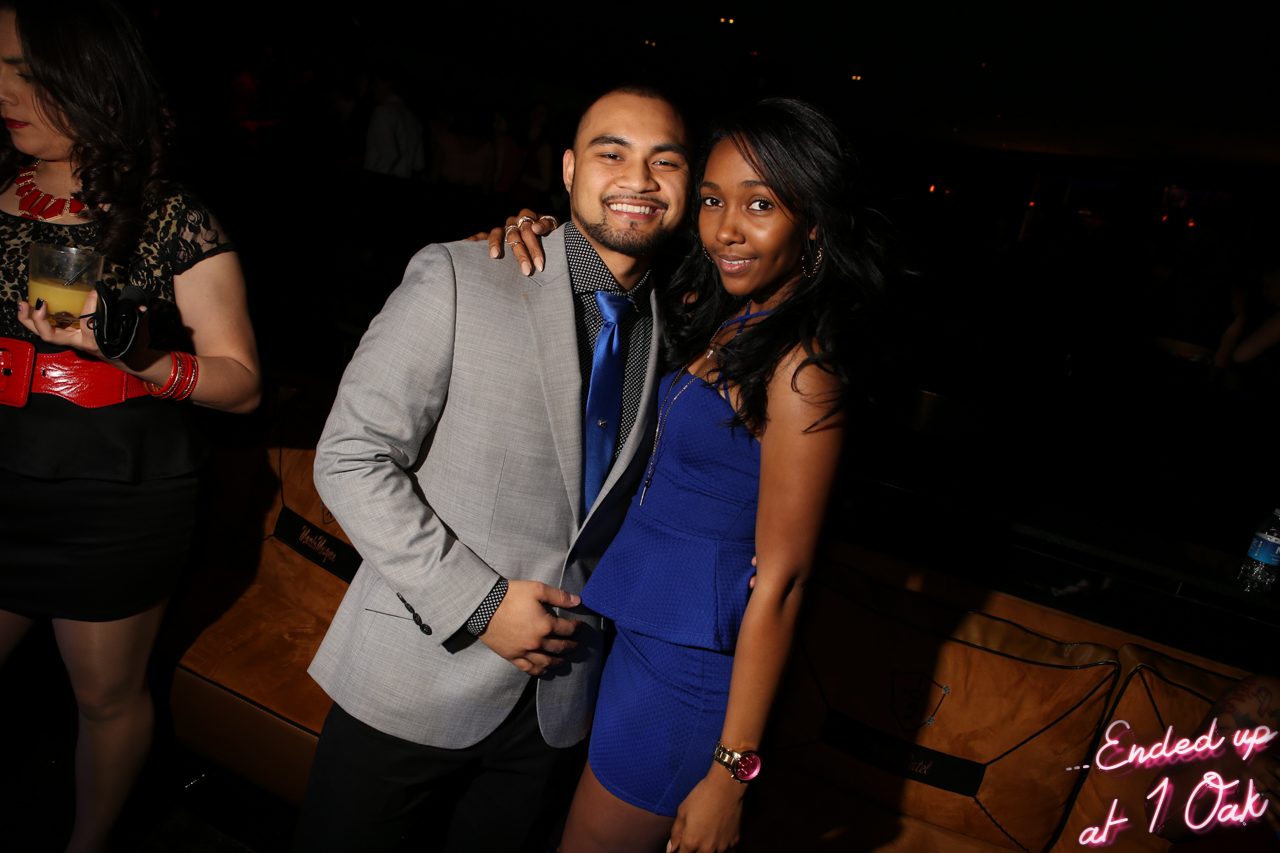In the image, a man and a woman are warmly hugging each other and looking forward, smiling. The man, who appears to be Mexican, is dressed in a grey suit with black buttons, complemented by a shiny blue tie. He has some facial hair and wears a collared shirt with white specks. The woman, who is black, is clad in a long, dark blue dress that reaches slightly past her shoulders, and she is wearing a watch on her wrist. They stand centered against a completely dark background dotted with points of light. To the left, a woman is holding a cup with a yellow liquid and looking down. On the lower left of the image, pink text reads "Ended up at 10 a.k.," while the lower right features the same pink and white text stating, "Ended up at One Oak."